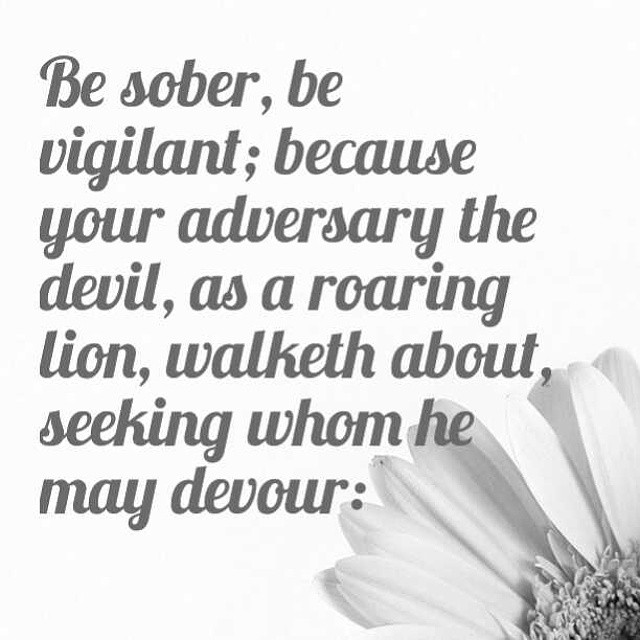This image is a monochromatic gray and white screenshot featuring an inspirational quote commonly found on social media platforms like Instagram or Pinterest. The quote, written in a sizable, elegant cursive script, reads, "Be sober, be vigilant, because your adversary the devil, as a roaring lion, walketh about, seeking whom he may devour;" with the concluding punctuation being a semicolon. The text is entirely in shades of gray, against a plain white background. In the bottom right corner, approximately a quarter of a sunflower, seemingly black and white due to the lack of color, is visible, showing part of its petals and center. The overall design is simplistic and typical of motivational posts often shared online.